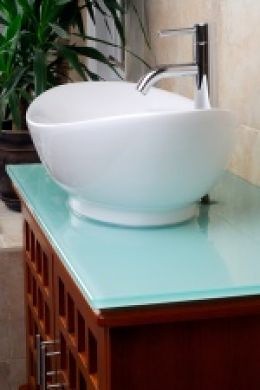This photograph captures a modern bathroom setup viewed from the side, focusing on a sink and cabinet arrangement. The sink is a large, white ceramic bowl with a cradle shape, complemented by a chrome faucet positioned at its rear. The sink rests on a strikingly pale blue, rectangular glass surface that tops a wood-grain cabinet. This cabinet features two front-facing doors with vertical, chrome-colored handles, adding a sleek touch to the natural wooden texture.

The cabinet is installed against a wall tiled with large, square ceramic tiles in a beige or creamy hue, adorned with subtle patterns of varying colors. In the background, a raised surface or bench is visible, hosting a pot plant. The plant pot is likely black or brown, creating a stark contrast to the vibrant, lush green foliage spilling out from it, enhancing the bathroom's refreshing ambiance.